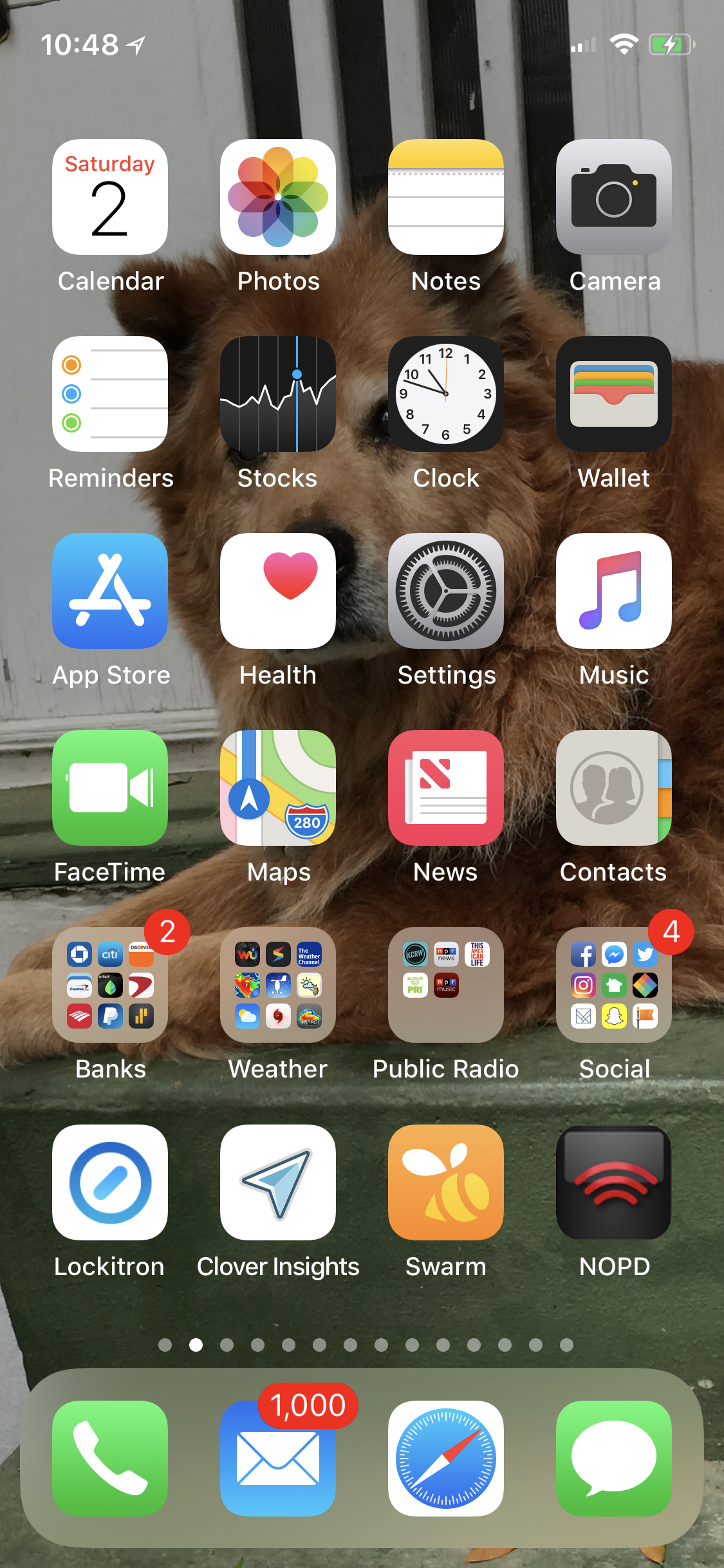This screenshot captures an iPhone home screen showcasing an organized array of apps against a personalized wallpaper. The background image is a charming photograph of the phone owner's dog, whose reddish-brown fur contrasts beautifully with the green stairs it is sitting on, highlighted by a white background.

At the top left of the screen, the time displays 10:48, and in the top right corner, the battery indicator is green with a lightning symbol, suggesting the iPhone is currently charging. 

The dock at the bottom of the screen holds four essential apps: Phone, Mail (with over a thousand unread emails), Safari, and Messages. 

The main screen is neatly arranged in a grid, starting from the top left:
1. Calendar
2. Photos
3. Notes
4. Camera
5. Reminders
6. Stocks
7. Clock
8. Wallet
9. App Store
10. Health
11. Settings
12. Music
13. FaceTime
14. Maps
15. News
16. Contacts
17. Banks (folder containing banking apps)
18. Weather (folder)
19. Public Radio (folder)
20. Social (folder)
21. Lockett
22. Clover
23. Insights
24. Swarm
25. No PD

The folders indicate categorized collections of apps for convenience, further emphasizing the user's meticulous organization of their digital space.